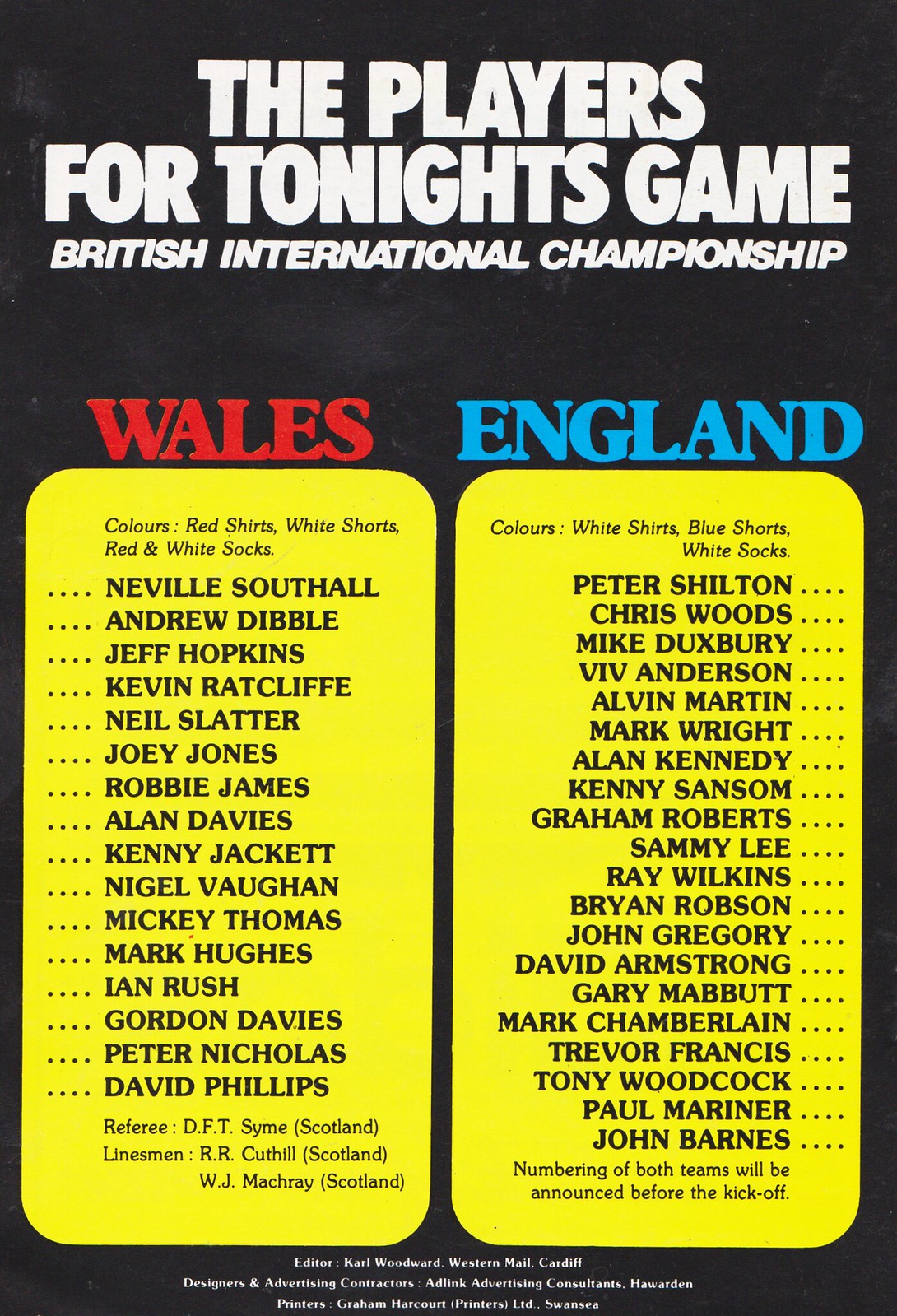The image features the front page of a magazine with a plain black background. Centered at the top in bold white text, it announces "The Players for Tonight's Game" followed by "British International Championship." Below this heading, there are two tall rectangles with beveled edges and bright yellow backgrounds. The rectangle on the left features the roster for Wales, labeled in red text, while the rectangle on the right showcases the roster for England, labeled in blue text.

For Wales, above the left rectangle, the label reads "Whales" in red print. Beneath it, in black print, are the team's colors: "Red Shirts, White Shorts, Red and White Socks." The player names listed are Neville Southall, Andrew Dibble, Jeff Hopkins, Kevin Ratcliffe, Neil Slatter, Joey Jones, Robbie James, Alan Davies, Kenny Jackett, Nigel Vaughan, Mickey Thomas, Mark Hughes, Ian Rush, Gordon Davies, Peter Nicholas, David Phillips. The officiating team includes referee DFT Syme from Scotland and linesmen RR Cuthill and WJ Mackay from Scotland.

For England, above the right rectangle, the label reads "England" in blue print. Beneath it, in black print, are the team's colors: "White Shirts, Blue Shorts, White Socks." The player names listed are Peter Shilton, Chris Woods, Mike Duxbury, Viv Anderson, Alvin Martin, Mark Wright, Alan Kennedy, Kenny Sansom, Graham Roberts, Sammy Lee, Ray Wilkins, Brian Robson, John Gregory, David Armstrong, Gary Mabbott, Mark Chamberlain, Trevor Francis, Tony Woodcock, Paul Mariner, John Barnes. The numbering for both teams was to be announced before kickoff.

At the very bottom, centered in white print, the magazine credits "Editor: Carl Woodard, Western Mail, Cardiff; Designers and Advertising Contractors: Adlink Advertising Consultants, Haywarden; Printers: Graham Harcourt, Printers LTD, Swansea."